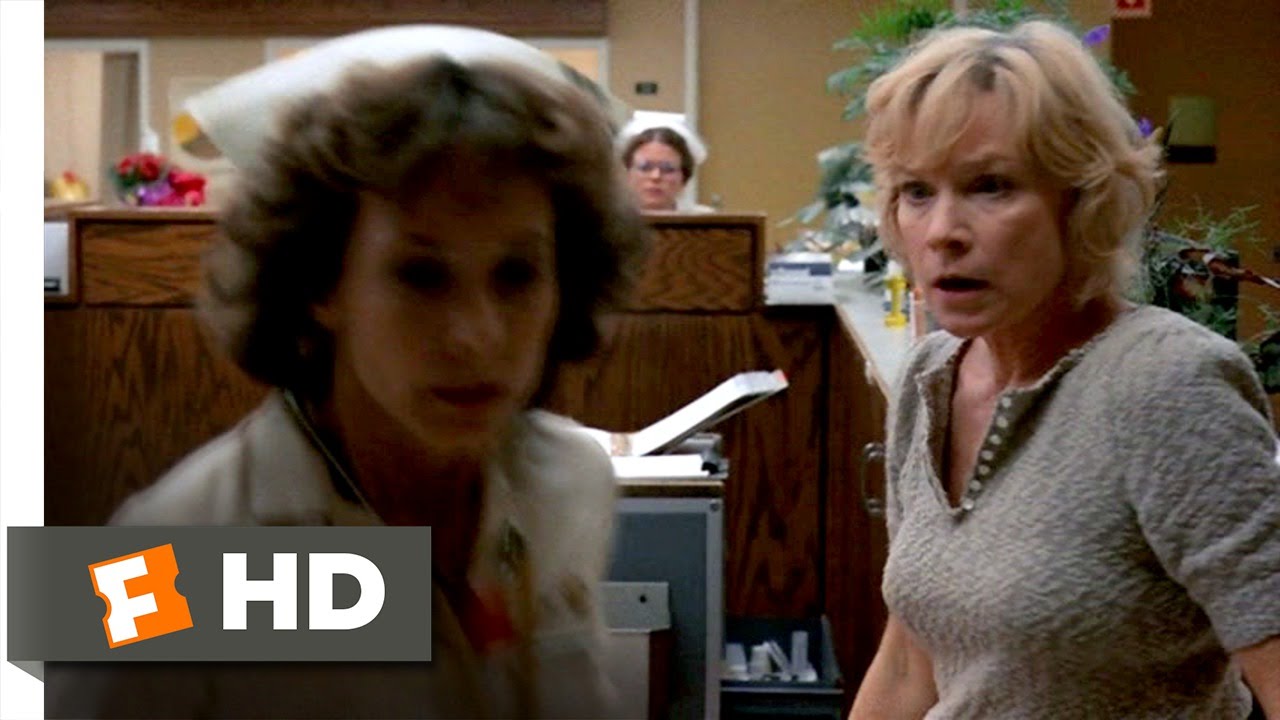This image appears to be a still photograph from a television show set in a hospital. In the foreground on the left side, there is a slightly blurred nurse with curly brown hair wearing a white headpiece and uniform. She is cut off at the chest and looks towards the right side of the frame. To her right, there is a shocked woman with short, blonde hair, dressed in a grey, v-neck top that appears to have buttons. She is also cut off at the waist and is gazing towards the nurse. Central in the background, behind a large brown desk or counter, another nurse can be seen wearing glasses and a white headpiece, but she is barely visible. To the left side of the image, a gray band containing a white letter "F" on an orange background and "HD" in white letters is visible. The background includes additional details such as medical machinery, a wastebasket, and a potted plant, enhancing the hospital setting ambiance.